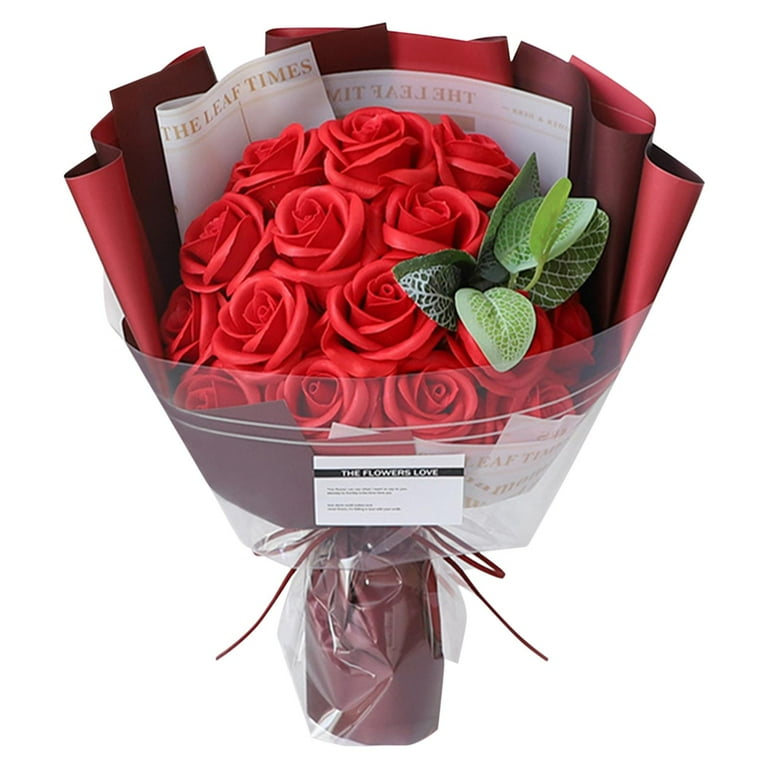This is an image of a vibrant bouquet of a dozen bright red roses, enhanced with some textured green foliage for contrast. The roses are wrapped in layers of deep burgundy and red paper, along with a piece of cellophane. The wrapping features a piece of white paper resembling a fake newspaper with the words "The Leaf Times" clearly visible. At the base, the bouquet is neatly tied together with a matching burgundy bow. There is a business card attached to the cellophane that reads "The Flowers Love," potentially the name of the company that crafted the bouquet. The overall presentation is meticulously detailed, giving the appearance of an artfully assembled, almost sculptural display.